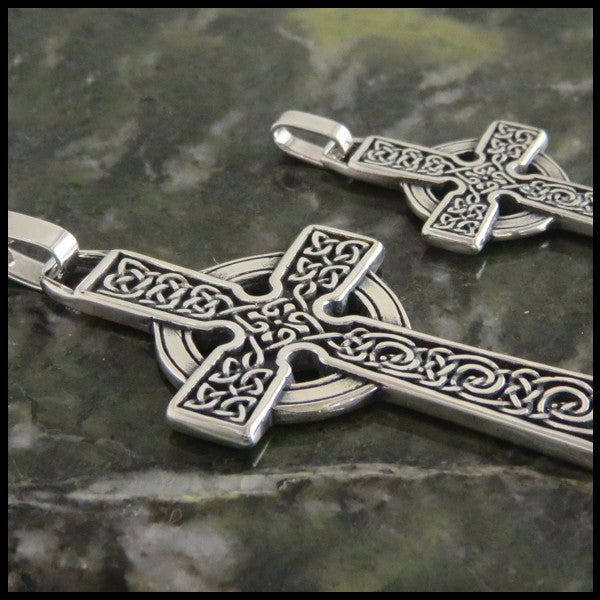This is a close-up photograph of two sterling silver crucifixes, potentially white gold, placed flat on a greenish-gray marble surface. The crucifixes are identical in design, featuring intricate etched patterns within the main part of the cross and a circular shield behind the arms of the cross. Each crucifix has a jeweler loop at the top, allowing them to be attached to a chain for use as a necklace. The larger crucifix is positioned centrally in the foreground, taking up most of the photo, while the smaller, identical crucifix is placed above and to the right of it. The detailed craftsmanship of these crucifixes is highlighted by the straight edges that taper inward at the intersection points, adding to their unique and elegant appearance.